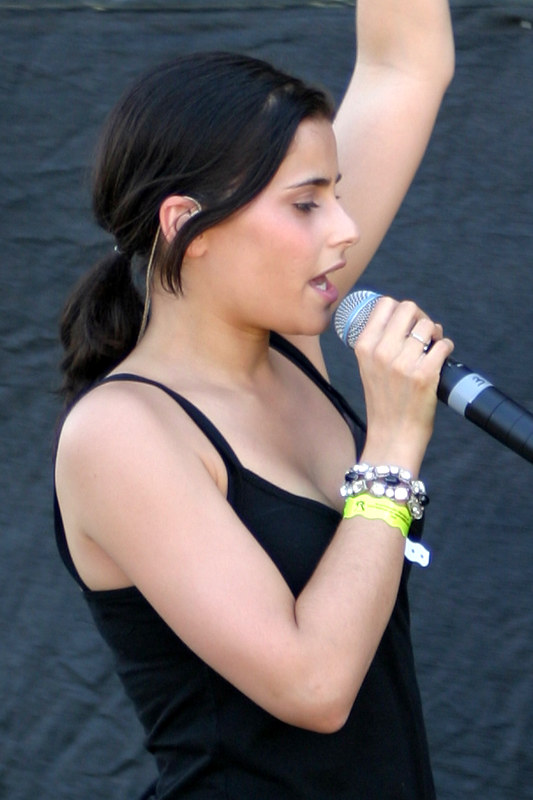The image captures a detailed profile view of a young woman in her early to mid-twenties, standing sideways against a dark, wrinkled curtain backdrop that appears to be green or brown. She has a lighter skin complexion and her black hair is tied back in a ponytail. An earpiece with a visible cord extends from her ear down her back. She is dressed in a black tank top and accessorized with multiple bracelets, including black and white beaded ones and a yellow or lime green entrance tag on her right wrist. Her right hand grips a microphone close to her mouth, and her left arm is raised high in the air, suggesting she is singing. The scene is brightly lit, emphasizing the clear details of her expressive stance.